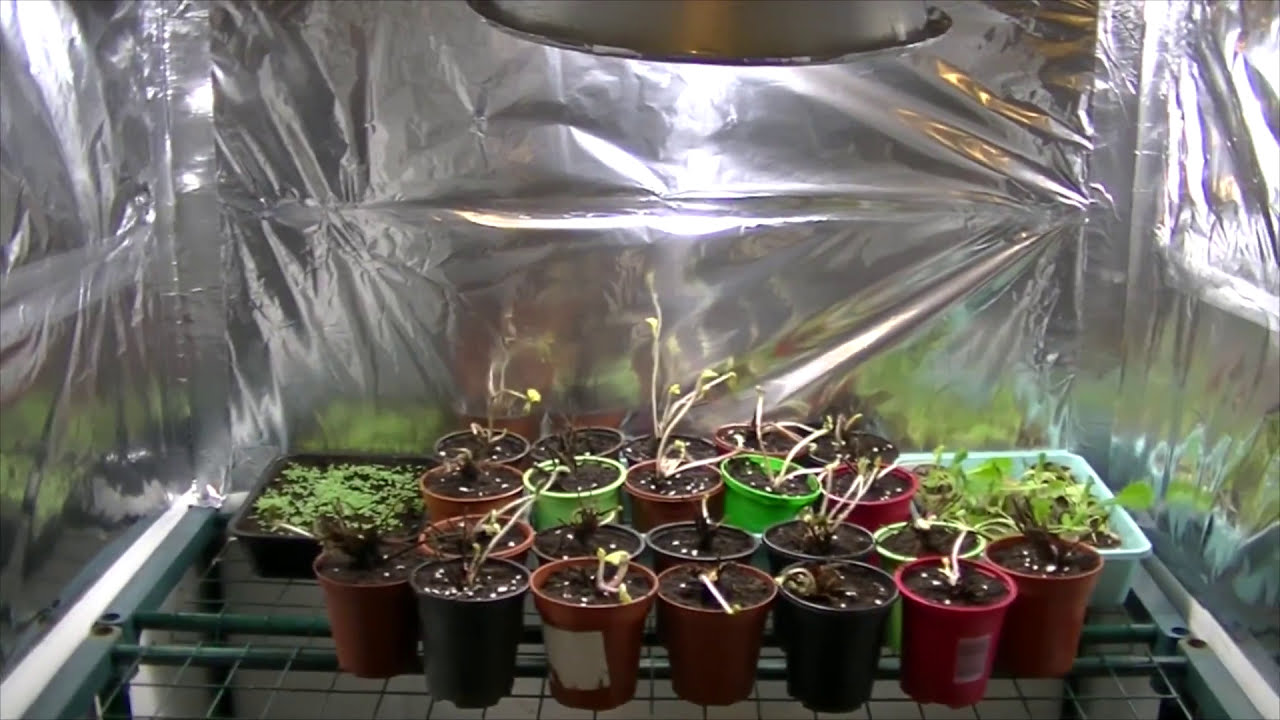The image showcases an indoor growing setup filled with various small potted plants at their seedling stage. These pots, made of different colored materials including red clay and neon green, are no more than a couple of inches tall and contain dark brown soil with young sprouts emerging. The sprouts feature white and reddish stems with tiny green buds and some leaves starting to form. The pots are arranged on top of a blue-painted grated metal rack, which provides support while allowing light and air to circulate.

Surrounding this central setup are larger trays of soil with green seedlings, positioned on the left and right sides. The entire area is enclosed in a temporary greenhouse structure composed of thick, opaque plastic sheeting with oval cut-outs that function as windows, allowing filtered light to penetrate. Additionally, the walls and back of the space are covered with reflective tinfoil, which helps to direct light uniformly onto the plants. Above the setup, a round metal grow lamp shines down, providing the necessary light for the seedlings to thrive. This meticulous arrangement ensures optimal growing conditions, emphasizing the importance of light and environment control for young plants.